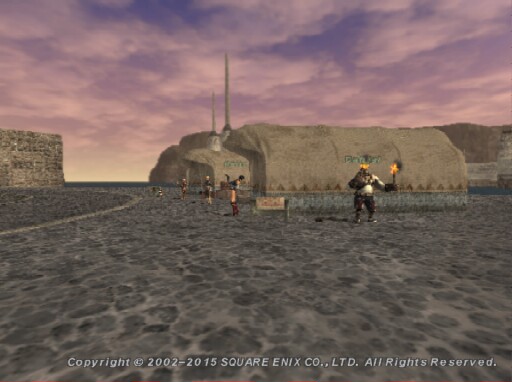In this image, which appears to be a screenshot from a video game developed by Square Enix (as indicated by the "Copyright 2002-2015 Square Enix Co." at the bottom), we are given a glimpse into a richly detailed fantasy world. The setting reveals a broad, open landscape that evokes either a desert or a medieval terrain, with the ground seemingly covered in a mix of rocks and dirt. The air is filled with a fantasy ambiance, emphasized by the purple sky adorned with swirling clouds. 

In the distance, several characters can be observed, albeit somewhat blurry. One prominent figure stands out due to its large size and the torch it holds, contributing to the game's mystical and adventurous atmosphere. This is further heightened by the presence of structures that resemble tents, faintly visible in the background. The overall scene conveys the essence of a fantastical realm, inviting players into a world of exploration and imagination.